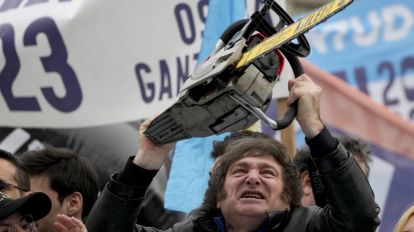In a brightly lit outdoor setting, a large crowd gathers, participating in what appears to be a rally or protest. The throng consists mostly of the tops of people's heads, but one man stands prominently at the forefront. He seems to be in his late 50s, wearing a gray jacket and a fur-lined cap, with brown hair peeking out. In his hands, he hoists a chainsaw skyward with a look of strained determination on his face. The chainsaw itself is distinctive, featuring a yellow blade encased in gray, with black handles firmly gripped by the man. Behind him, various colorful banners and posters, in shades of blue, white, and salmon, are held aloft by other protestors, though their texts are mostly indiscernible. The scene is rich with the tension and fervor of a public demonstration.